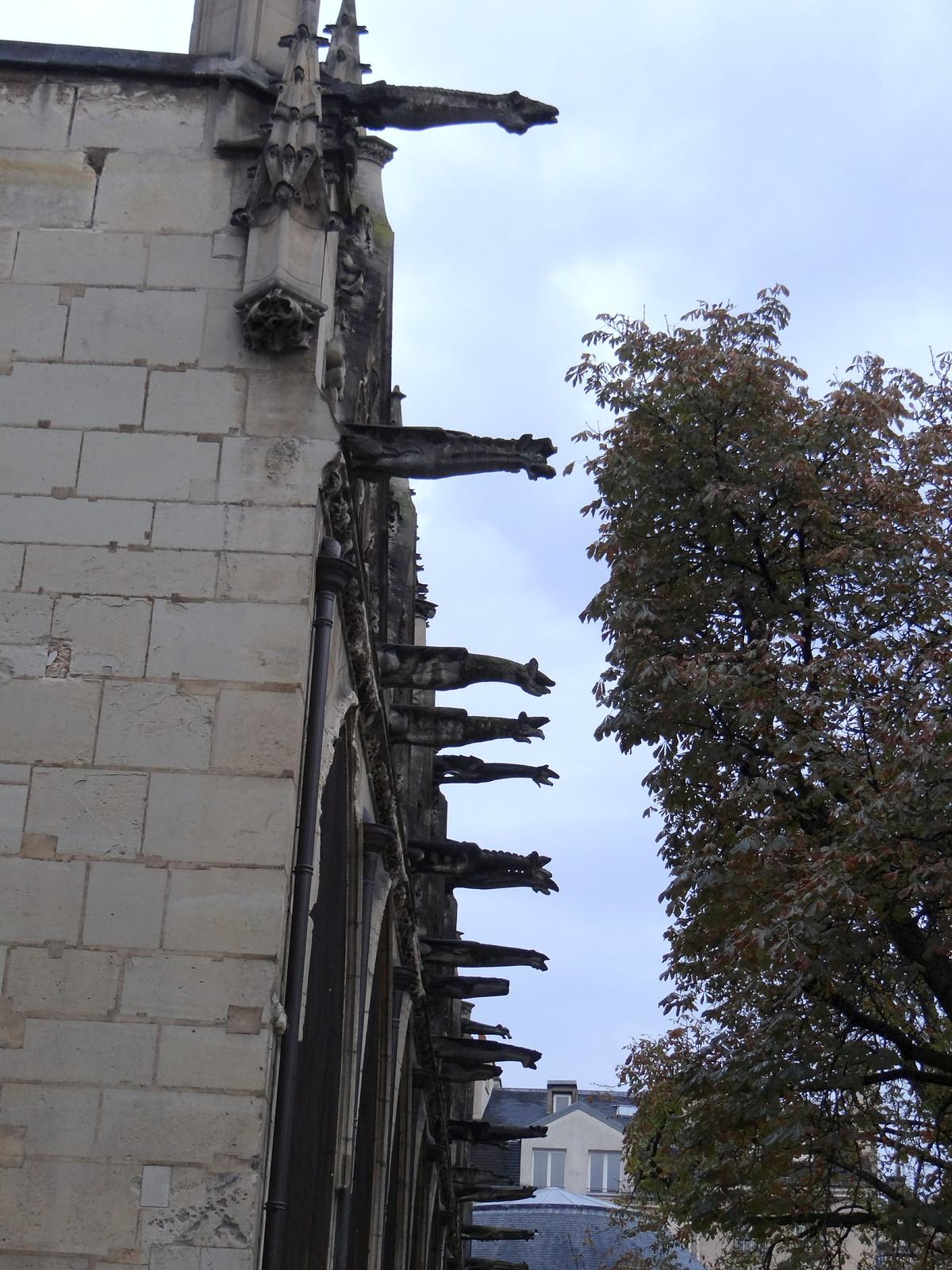This photograph captures the side of a grand cathedral, characterized by an array of architectural details. The building is constructed from a mix of light beige bricks, unevenly sized, with brownish-beige putty filling the gaps. The wall on the left side of the photograph is adorned with multiple stone sculptures protruding dramatically from the building's façade. These sculptures, resembling hands or mythical creatures, are likely water spouts, each about two to three feet long, with mouths that channel rainwater away from the structure. 

Below these sculptures, a series of large, dramatic, rounded doorways can be seen, framed by pillars that converge towards a vanishing point in the center of the image. The building's black roof, adorned with a partially visible tower, adds to the gothic aesthetic. 

In the background, the sky is cloudy and dark, casting a somewhat moody atmosphere over the scene. A large tree occupies the right half of the photograph, its leafy branches extending prominently upwards. Farther in the distance, a two-story residential building with a black roof and beige walls, and a visible tent or tower in front, can be seen. The entire scene is enveloped in the somber tones of a cloudy day, enhancing the cathedral's imposing and historical presence.